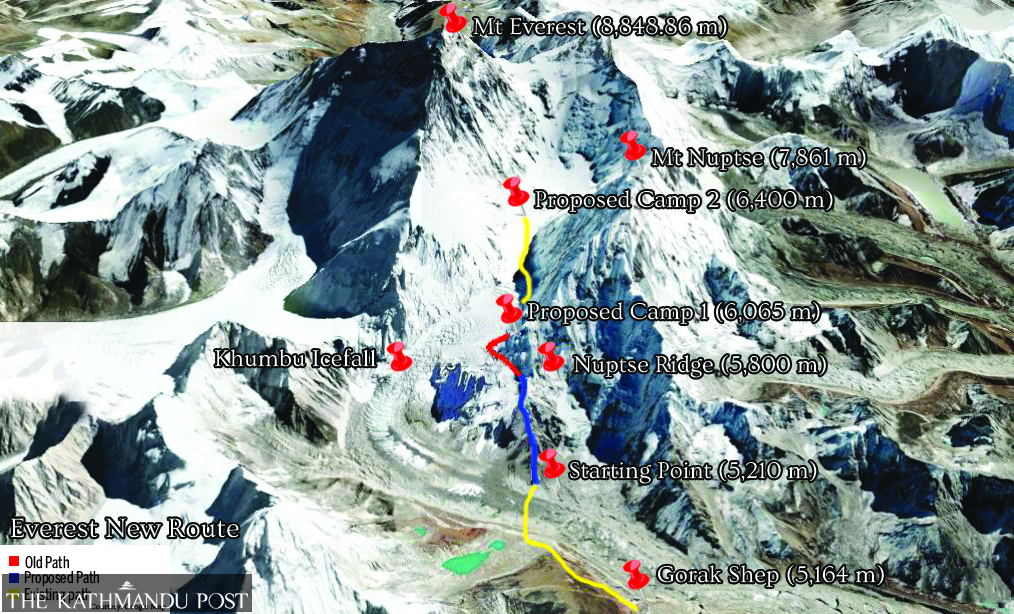The image is a highly detailed, top-down satellite view of Mount Everest and its surrounding peaks, illustrating different climbing routes and key locations. The legend in the bottom left corner indicates route types: red for the old path, blue for the proposed new path, and yellow for an estimated path. This map is credited to the Kathmandu Post.

At the top center of the image is Mount Everest, standing at 8,848.86 meters. Just below it is Mount Nuptse, which reaches 7,861 meters. Further down, the proposed Camp 2 is marked at 6,400 meters, connected by a yellow path. Below that is the proposed Camp 1 at 6,065 meters, which is intersected by the old red path. To the left, you can see the Khumbu Icefall, while the Nuptse Ridge, at 5,800 meters, is on the right.

In the lower part of the image, a blue path trails downwards to the starting point at 5,210 meters. Nearby, Gorak Shep is indicated, standing at 5,164 meters. The image is predominantly of snow-covered mountain terrain, with colored paths and cartoonish pushpins marking significant locations and elevations.